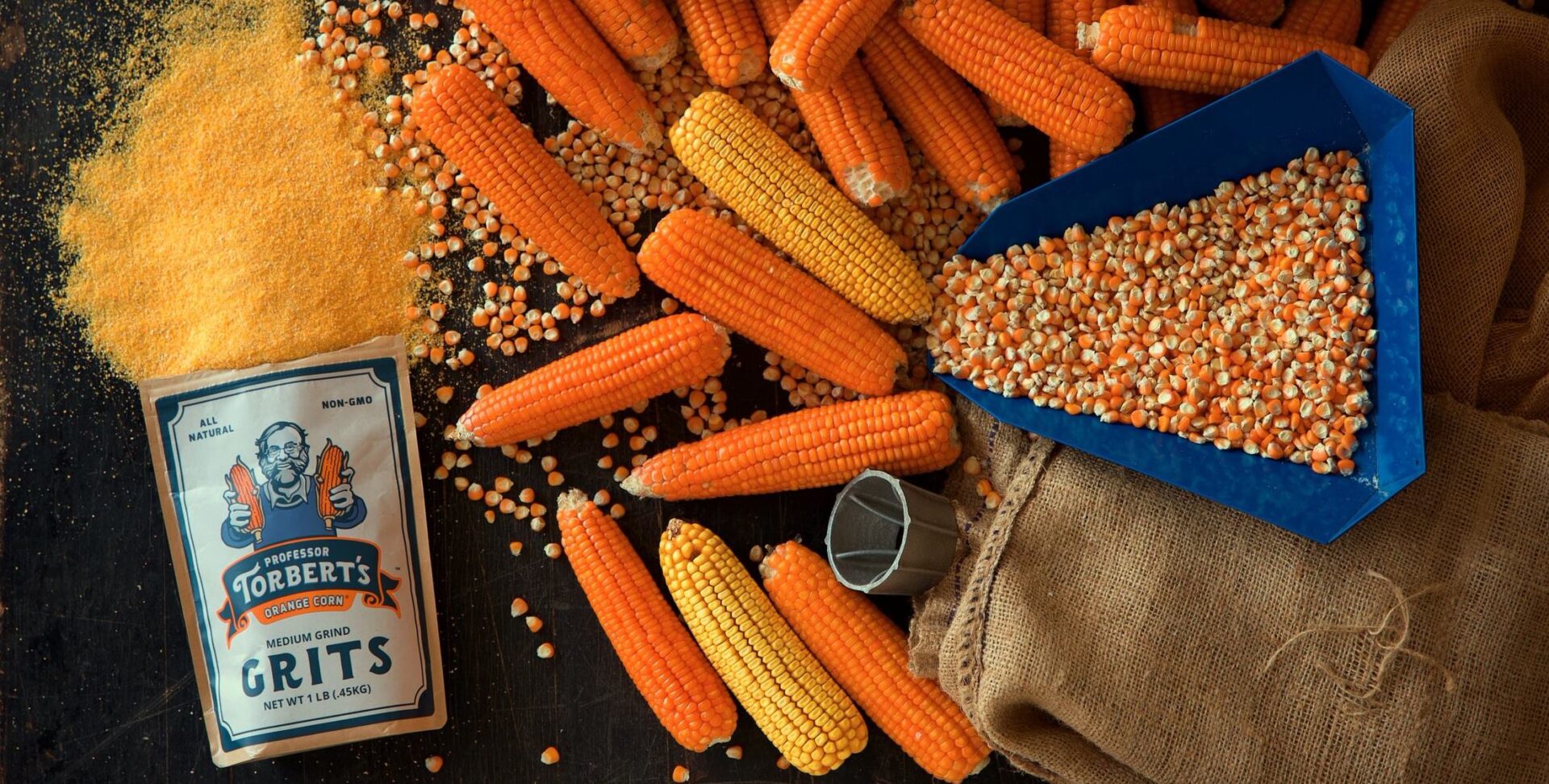The photo, taken indoors, features a black wooden table as the background. Dominating the right side of the image is a blue, diamond-shaped bowl filled with dried corn kernels, resting on a brown burlap sack. Adjacent to this, an array of corn cobs stretches from the top right to the bottom middle of the frame, showcasing a striking mix of bright orange and traditional yellow hues. On the left side, a brown rectangular package with a white label catches the eye. This is a bag of Professor Torbert's Orange Corn Medium Grind Grits, with a picture of a man clad in blue holding two corn stalks. The bag's contents, an orange-hued powder, spill out onto the table, further emphasizing the vibrant palette of the scene. To the left of the corn cobs lies an orange plastic scooper, also filled with orange corn, adding to the composition's rich display of colors and textures.